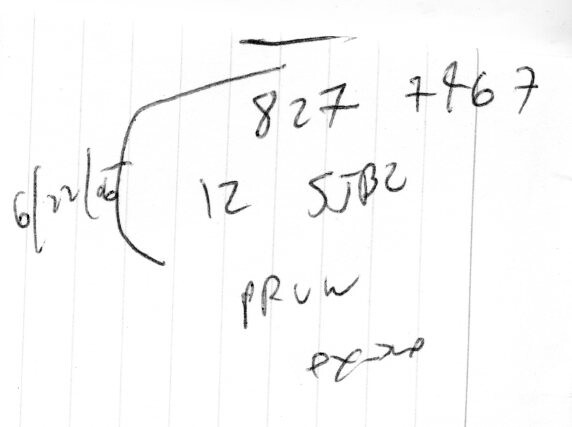This photograph captures handwritten text in black ink on a white, lined paper. The lines on the paper are gray. Notably, in the top section, there is a sequence of numbers: "8277967". Below, there is another number, "12", followed by a somewhat illegible string that could potentially be "SJB2". Further down, the letters "PRUW" are clearly written. The bottom section features some ambiguous squiggles, making it difficult to discern any specific characters or shapes.

A prominent black line runs across the top of the paper, serving no apparent purpose related to the writing. In the lower portion of the document, an encircling line encompasses additional text that includes the written date "6-22-06". There may be other writings on the page that are not fully visible in this photograph.